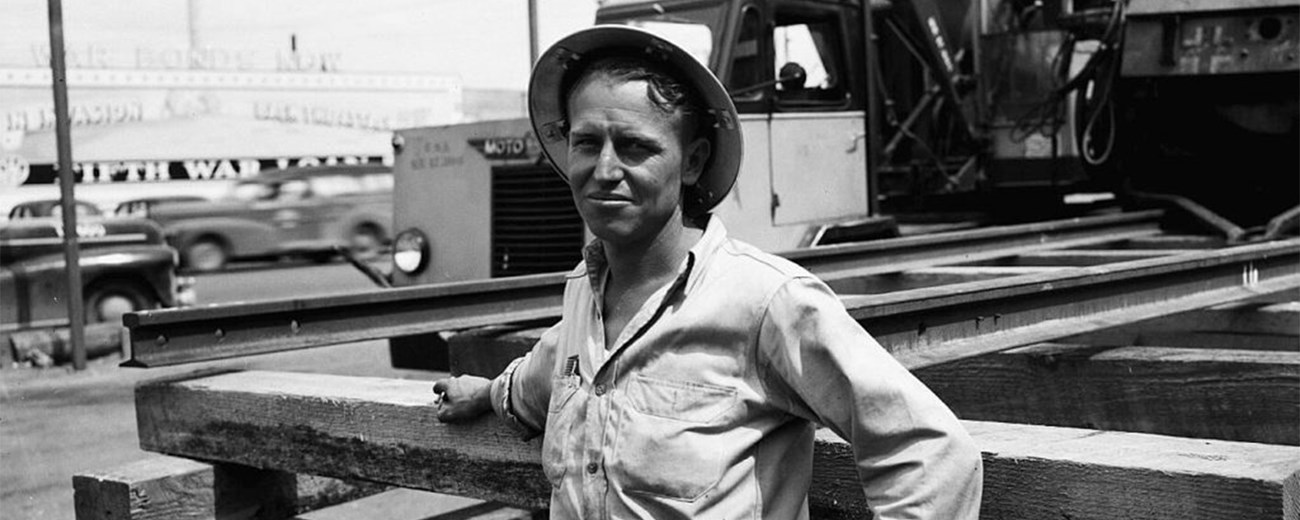This black and white photograph captures a long-faced individual standing outside on what appears to be a construction or work site. They are dressed in a light-colored, long-sleeved, buttoned shirt with chest pockets and wearing a distinctive round, circle-edged hat. The person has a somewhat frowning or squinty expression, possibly attempting a smile, and leans back on a wooden beam with a metal rod across it, extending their right hand over the beam. Behind them, there is a white panel, possibly part of a truck, with the word "Moto" visible on the front. In the background, to the left side, old-fashioned cars reminiscent of the 1950s can be seen driving by. On the right side of the image, there's a darker area with industrial equipment, including concrete and metal beams. The backdrop features a partial advertisement reading "Fifth War," and hints of a cityscape lining above it.